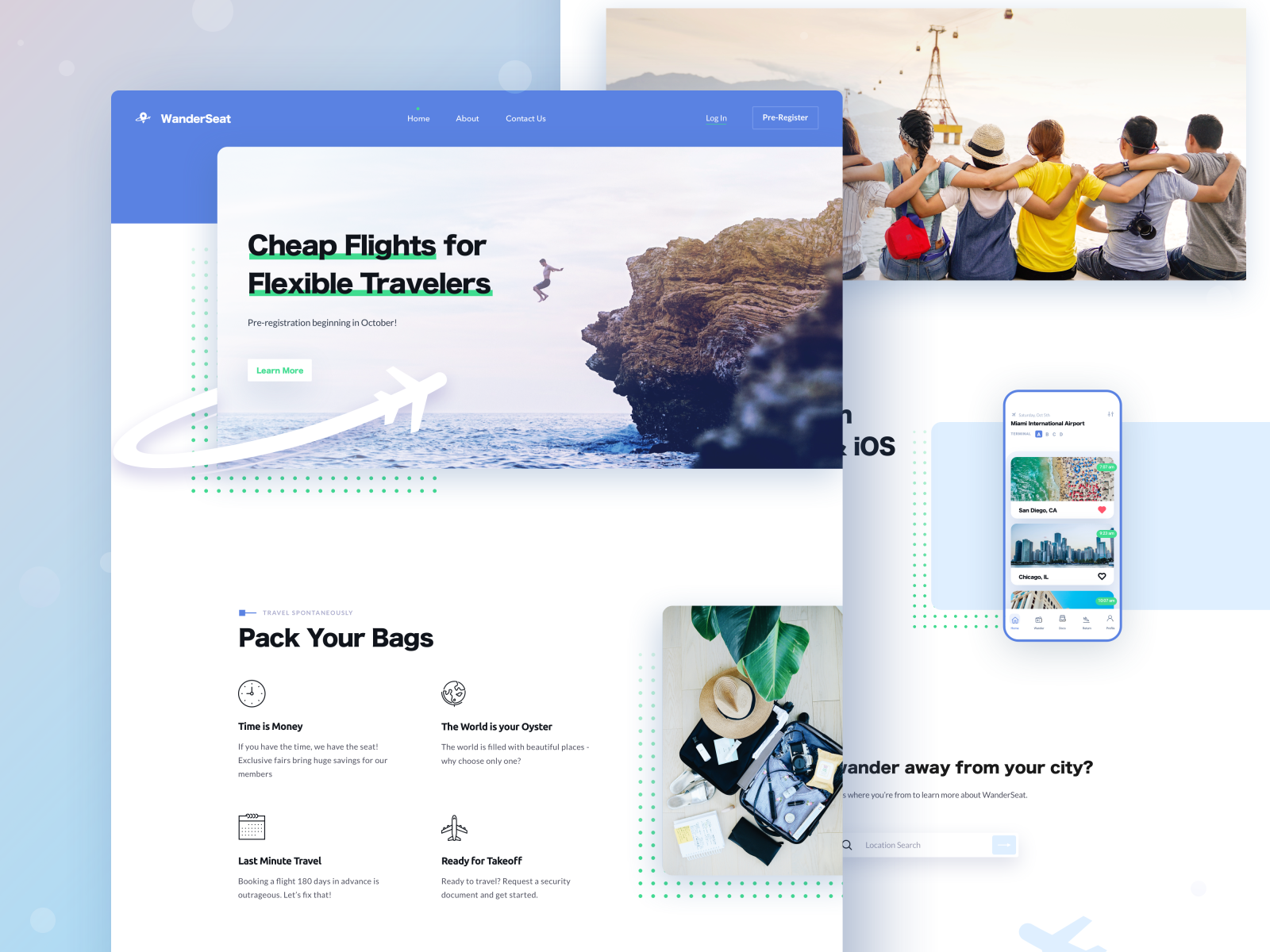This screenshot captures the homepage of the "Wonderseat" website, characterized by its blue header that includes options to log in, register, and navigate various sections. Below the header, there's a prominent banner image featuring text that encourages "Flights for Flexible Travelers." A graphic of an airplane superimposed over a picturesque scene of a person cliff diving off a mountainside adds a sense of adventure, further enhanced by decorative graph dots. 

Underneath the banner, the section titled "Pack Your Bags" outlines four focal points: a clock icon paired with "Time is Money," suggesting the importance of efficiency; a globe icon with "The World is Your Oyster," emphasizing limitless travel opportunities; an airplane icon representing travel logistics; and a comprehensive packing guide. To the right, an image illustrates a neatly packed suitcase complete with clothes and a hat. Adjacent to it, a cell phone display indicates the availability of a corresponding app, reinforcing the website's user-friendly, resourceful nature.